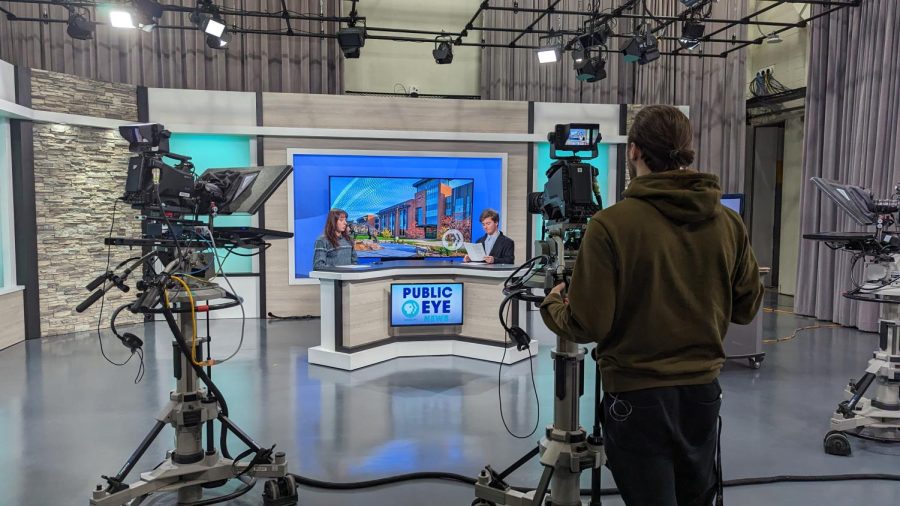The photograph showcases a newsroom soundstage for a local PBS show called "Public Eye." The rectangular image, wider than it is tall, captures a detailed scene from behind one of the cameramen. This cameraman, positioned toward the front of the picture, is wearing a brown hoodie, black pants, and has his brown hair tied back in a bun. He is operating a camera, and another camera is visible beside him. 

At the center of the image, a screen displaying "Public Eye" in blue is prominent, with a PBS logo potentially visible. Two newscasters are seated at a desk in front of this screen, featuring a blue background with drawn buildings. The male newscaster on the right holds a white paper, seemingly checking the news, while the female newscaster on the left looks over at him.

The set is surrounded by various stage equipment, including black metal rigs and lights, which are visible high up in the background. The staged area where the newscasters are seated is about six feet tall, emphasizing the compact but professional setting. The overall scene captures the hustle and bustle of a live newsroom environment, with intricate details of both the set and the behind-the-scenes activities.